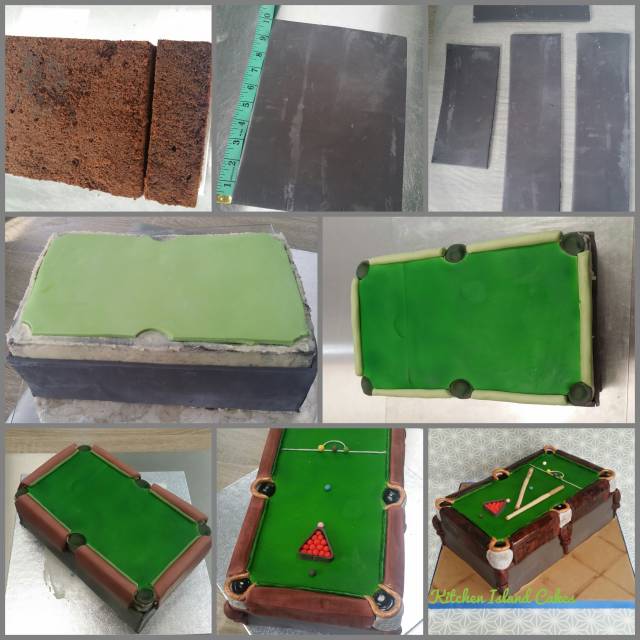This image is a detailed montage of ten photographs that illustrate the step-by-step construction of a pool table. The top row of three photographs highlights the raw materials: the upper left image shows a dark brown brick-like material, likely composite wood; the middle image features a slate-colored material, measured to be 10 inches long, and the upper right image shows four slate sections, with two longer than the other two. The middle row, consisting of two images, showcases the assembly process: the left photo displays the initial framework with green felt being laid on top, and the right photo shows further progress with the frame being more defined and the felt tailored to fit the table. 

The bottom row of three images reveals the finishing touches. The left image depicts pool tables with green felt and some brown wooden borders, the middle image focuses on a nearly complete pool table with a set of red balls racked and aligned pockets, and the right image presents the final product, featuring a fully constructed pool table equipped with racked balls, cue sticks, and various accessories scattered on top. Interestingly, within the bottom-right photograph, there is a caption that reads "Kitchen Island Cakes," although its connection to the pool table construction is unclear. Overall, this montage provides a comprehensive visual narrative of transforming raw materials into a finished pool table.